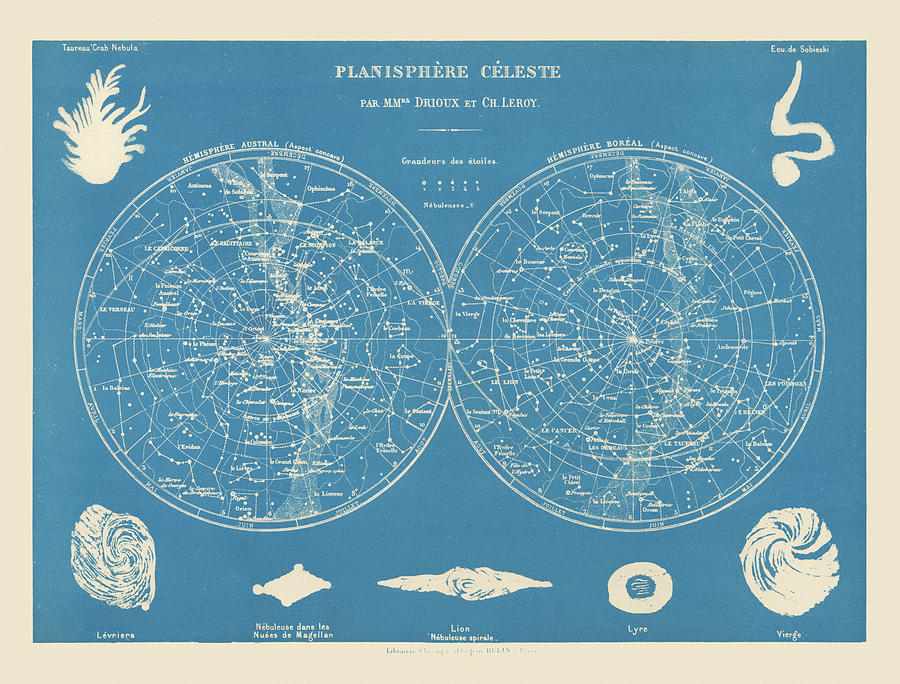The image appears to be a detailed vintage-style celestial star map with a predominant baby blue background and intricate white text and illustrations. It features two main overlapping circles, resembling an infinity symbol, labeled "Hemisphere Astral" on the left and "Hemisphere Boreal" on the right. Each circle is adorned with latitude and longitude lines, intersecting white lines, and numerous white dots likely representing stars and constellations. Notable constellations such as the Big Dipper and possibly Virgo or Sagittarius can be identified among the intricate patterns.

At the top center of the image, the title "Planisphere Celeste" is exquisitely displayed, followed by a secondary line of smaller, less legible text. Surrounding the circles are seven distinct graphical elements: in the upper left and right corners, there are abstract patterns—one possibly representing a fingerprint and another resembling a swirling design. The bottom of the image showcases additional symbolic designs: on the left is a shape akin to a fingerprint, the center features a leaf, and towards the right, there is a diamond and what appears to be an avocado pit or seed.

Overall, the image has a decorative beige border framing the detailed celestial illustration, evoking the aesthetic of an old astronomical chart or diagram.